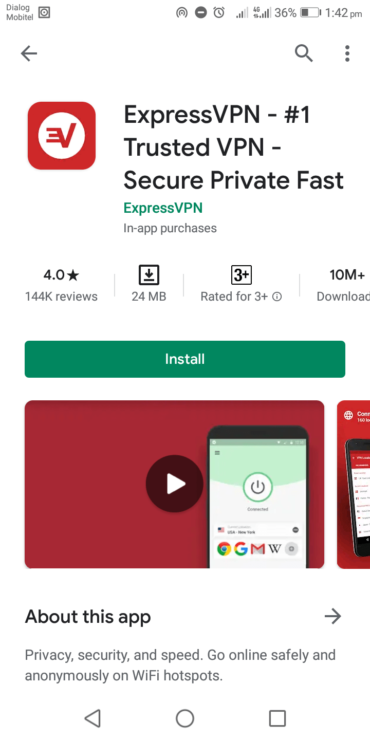The image depicts a digital device screen displaying the "ExpressVPN" application details. At the top of the screen, there is a "V" inside a circle, and another "V" followed by an "E" next to it, which are all enclosed within a red square. The header reads "Digital Dialogue Mobitel," and at the very top-right corner, essential status indicators are shown: a clock reads "1:42 PM," the signal strength is presented with three bars, and the battery level is at 36%.

Beneath this header, there are user-interface elements including a black back arrow, a search icon, and three vertical dots (options menu). The main section of the screen is dedicated to the ExpressVPN app details. The description reads: "ExpressVPN: Number One Trusted VPN - Secure, Private, Fast." Underneath, in green text, "ExpressVPN" is displayed again, followed by "In-app purchases" in black text.

The app boasts a rating of four stars from 144K reviews. It is a 24 MB download, rated suitable for ages 3+, and has over 10 million downloads. The "Install" button is prominently highlighted in green. Below the install button, a video thumbnail with a red background and an image of a phone is presented, available for playback. Additional app information includes, "About this app: Privacy, security, and speed. Go online safely and anonymously on Wi-Fi hotspots."

At the very bottom of the screen, the standard navigation icons are visible: a back arrow, a circle, and a square.